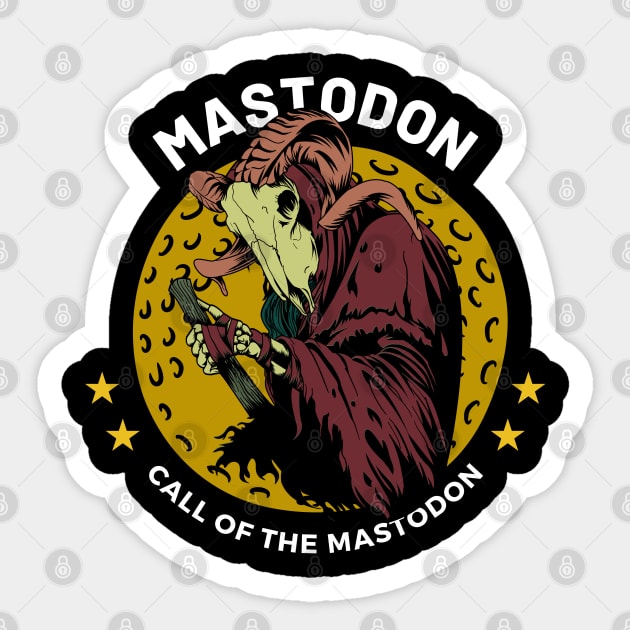The image is a sticker featuring a logo for "Mastodon" with the text "Mastodon" at the top and "Call of the Mastodon" at the bottom. The sticker is slightly circular with portions extending out on the top, left, and right sides, and has a white outline with a black interior. At its center, against a dark yellow background, is a striking character design: a skeletal figure with a ram's skull for a head, complete with a curving horn. The figure is draped in a maroon or burgundy-colored robe and has long, bony arms and hands. The background also includes a crescent moon shape, along with scattered stars on the left and right.